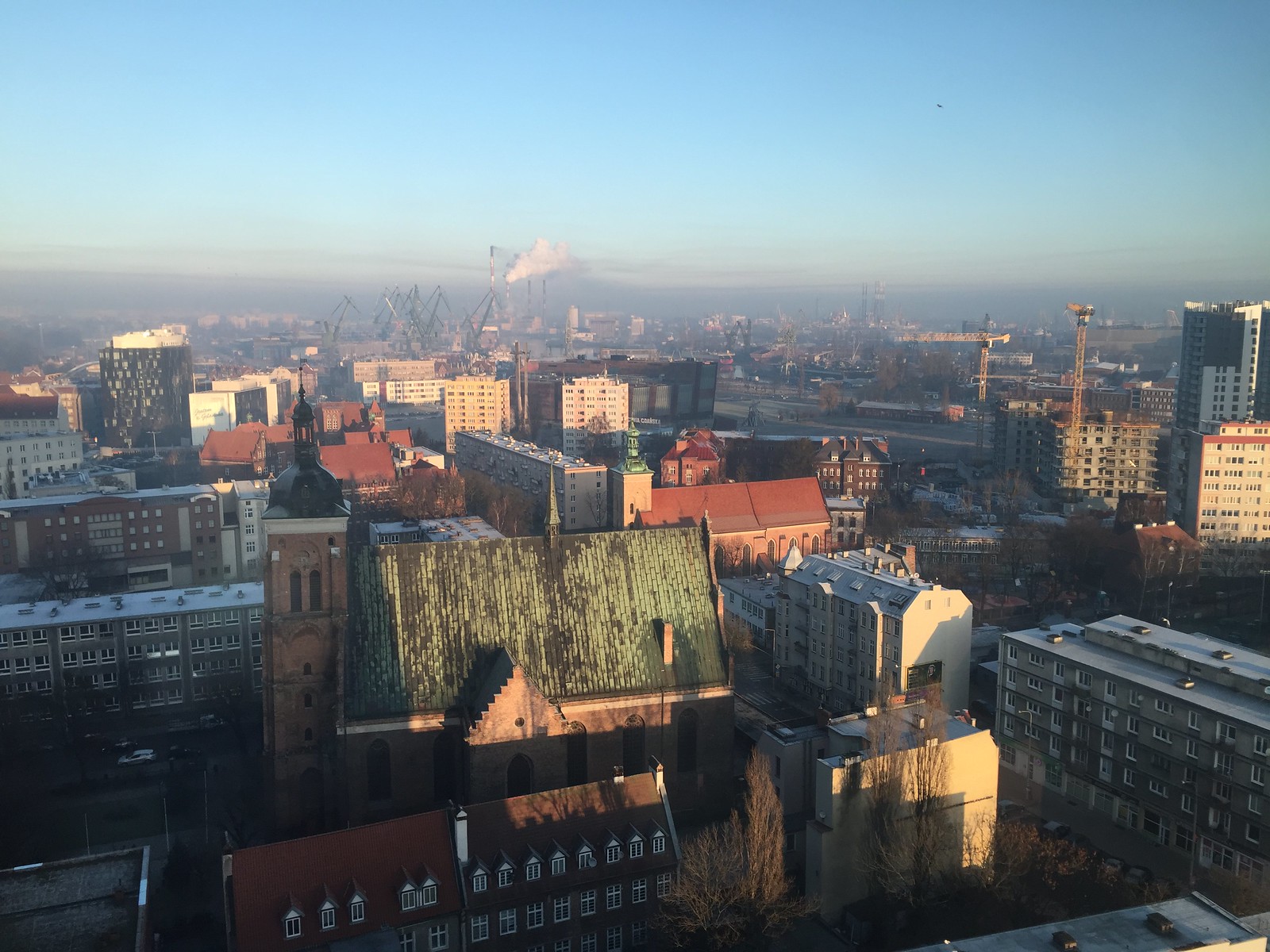From a high vantage point, this outdoor image captures a bustling cityscape sprawling beneath a clear, bright blue sky. The scene is dominated by myriad buildings, roughly three dozen in total, ranging from brown brick structures with white windows to larger, older buildings with distinctive features. Notably, there’s a prominent stone building with a green roof, showing signs of weathering with green and brown patches. A standout feature in the middle of the frame is an older church made of red brick, crowned with a faded copper roof. The foreground and midground are peppered with streets lined with sparse traffic and trees stripped of their leaves, suggesting a fall setting. In the distance, the city's industrial side reveals itself with several smokestacks emitting smoke into the sky. Beyond, a mountain capped in snow rises against the horizon, adding a serene touch to the otherwise dynamic urban tableau. The entire scene is bathed in natural sunlight, creating a lightly shadowed, time-stilled representation of a calm, yet lively city.